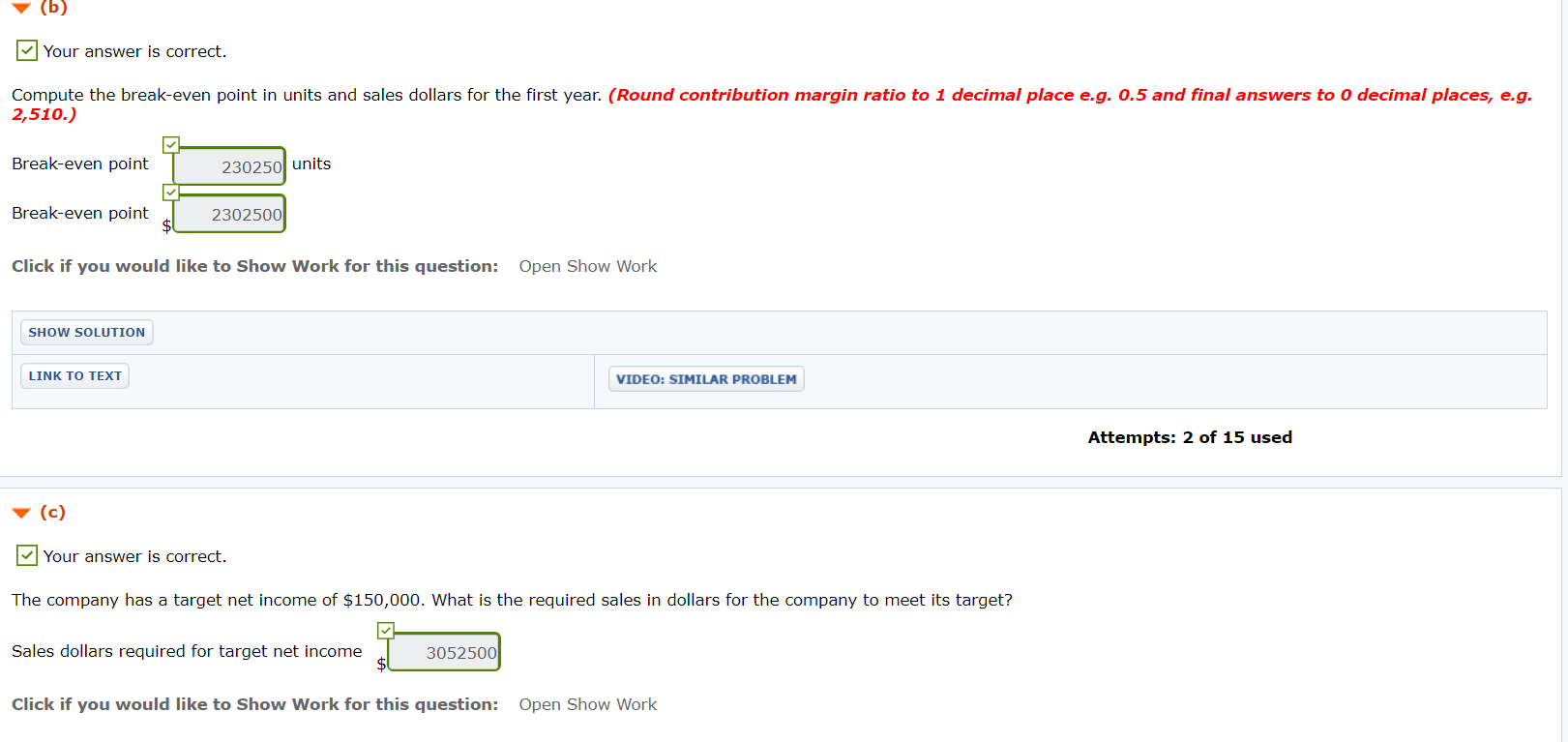In the image, a computer screen is displayed featuring a detailed break-even analysis interface. At the top of the screen, the letter "B" is enclosed in parentheses. Directly beneath this, the text "Your answer is correct" is prominently shown. The subsequent line, in red text, reads: "Calculate the break-even point in units and sales dollars for the first year. Round contribution margin ratio to one decimal place, e.g., 0.5. And final answers to zero decimal places, e.g., 2,510."

Below this instructional text, there are two green rectangles. The first green rectangle displays the break-even point in units, and the second green rectangle shows the break-even point in sales dollars. Following these values, a prompt in black text states: "Click if you would like to show work for this question." 

Continuing downward, there are three very small rectangles featuring blue text. Positioned to the right of these rectangles, the black text states: "Types 2050-used." Below this, the letter "C" appears, accompanied by the statement "Your answer is correct."

Subsequent to this validation, a smaller font text reads: "Your company has a target net income of $150,000. What is the resulting sales in dollars for the company to meet this target?" This is followed by another green rectangle containing the necessary sales dollar amount to achieve the target net income.

At the very bottom of the screen, a final prompt in black text reads: "Click if you would like to show work for this question" and the option "Show work." The entire interface is set against a clean white background.